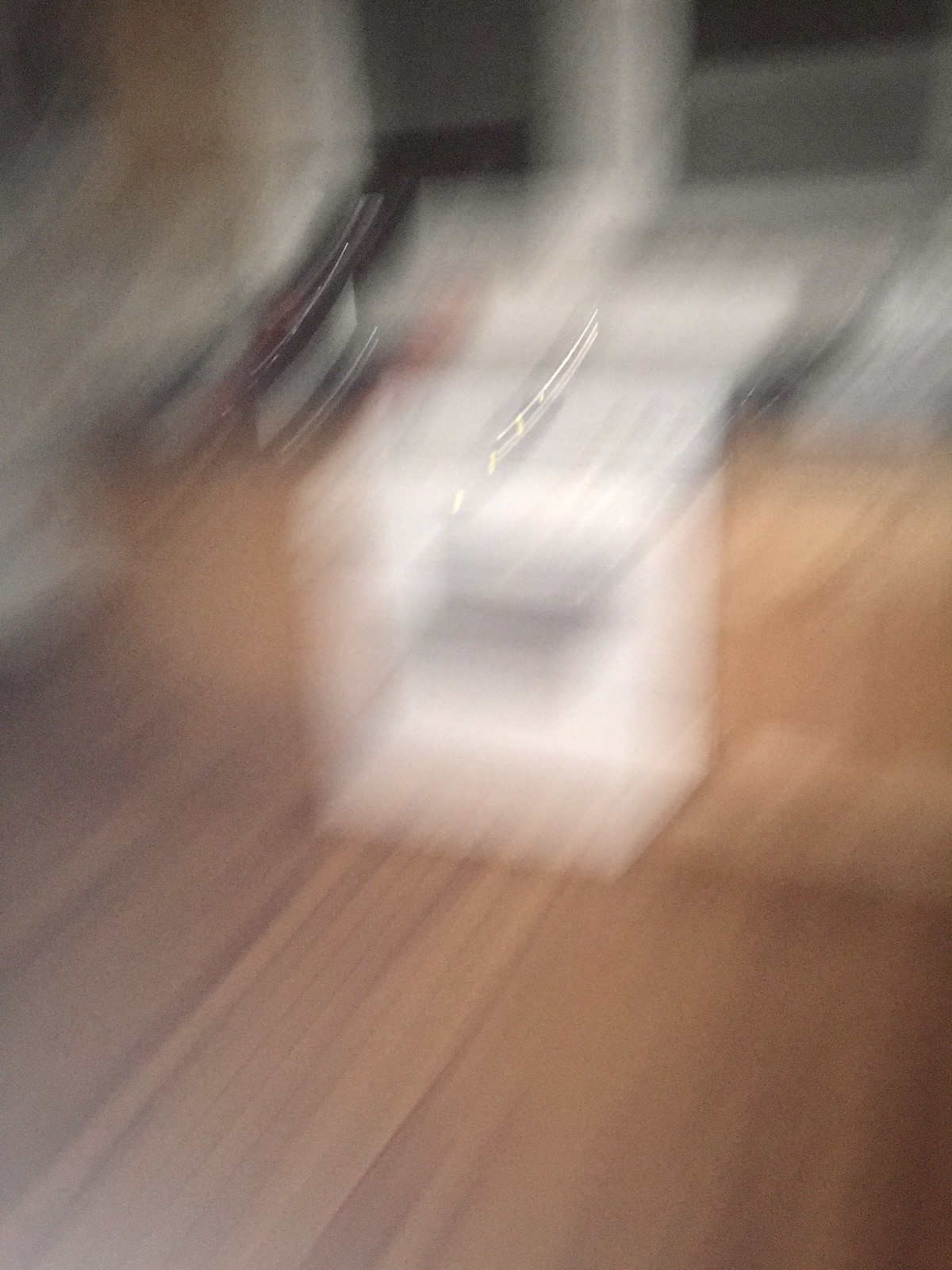The image is a very, very blurry color photograph, likely taken from a fast-moving camera due to the texture indicating movement. Despite the blurriness and dim lighting, we can discern that the scene is of a kitchen. Centered in the image is a white appliance, most likely a stove, as indicated by the darker rectangular area which resembles an oven door. Flanking the stove are two countertops with black surfaces, one on each side. Additionally, above the stove are two pairs of windows with white frames; one of the windows appears to be an older style crank window, while the other looks like an up-and-down shutter style. The kitchen floor is a nicely polished hardwood, adding a warm element to the ambiance. Above the stove, there is a small light fixture. The back wall partially reveals what seems to be a concrete surface. Though the photograph doesn't provide clarity on smaller countertop details, the overall impression is of a cozy kitchen space with a mixture of modern and vintage elements.